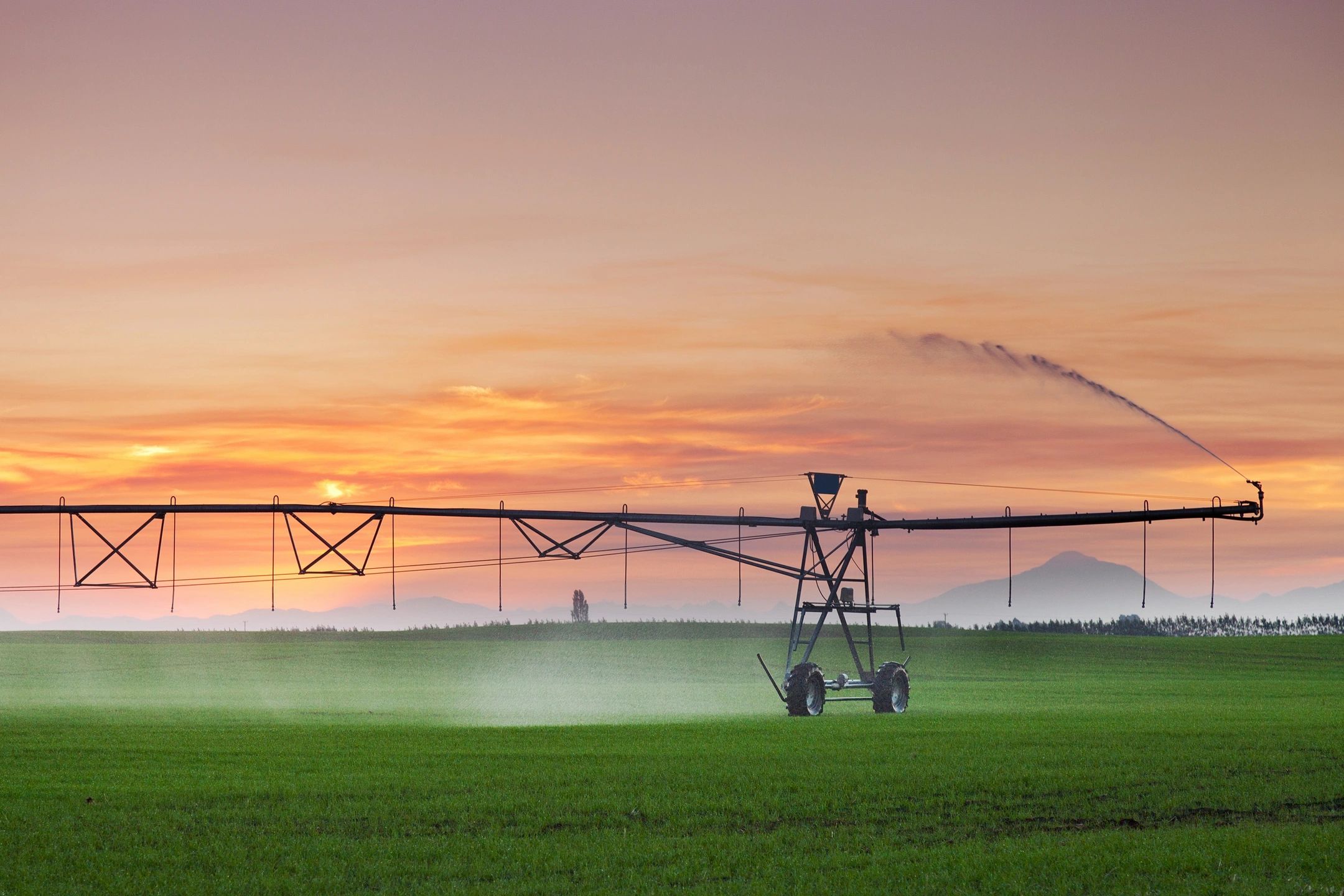This image captures a serene farm scene at sunset, where the sky is a beautiful blend of orange and yellow hues, lightly veiled by clouds. The foreground showcases a lush, expansive field of green crops that stretch across the frame, indicating their early stage of growth. Central to the image is a large irrigation system, propped up by wheels and extending across the middle of the field. Water is visibly spraying out from various nozzles, including one prominently at the end of the long rod, casting a mist over the crops. The scene is further framed by a distant, misty mountain range, adding depth and a sense of location to the quiet, natural beauty of the farmland.